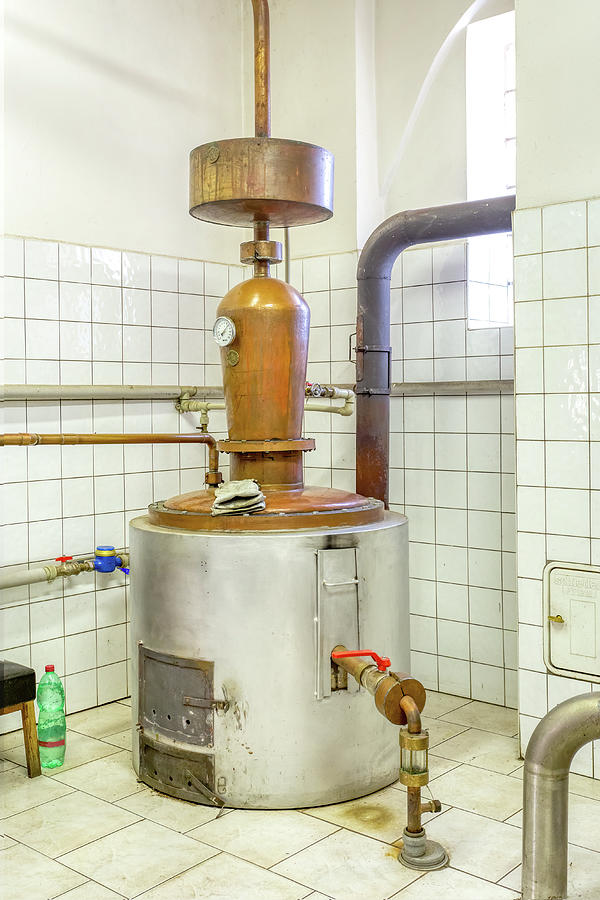The photograph depicts a still, typically used for distilling liquor, situated in a white-tiled room with glossy square ceramic tiles on the walls and floor. The room appears clinical and well-illuminated, suggesting a professional or industrial setting. The still itself is constructed from copper and features various gauges, including a prominent pressure gauge, as well as an array of complex tubing and valves intended for fluid transport. Attached to the bottom of the still is a door, likely for temperature adjustment, and a pair of gloves rests on top of the apparatus. To the left, part of a low bench is visible, holding a plastic jug of liquid. The setting is punctuated by the presence of industrial-type piping along the walls and a stool, possibly covered in black, positioned near a bottle of soft drink, such as Sprite. The overall color scheme is dominated by whites, silvers, and copper tones, lending to the room's sterile and utilitarian ambiance.